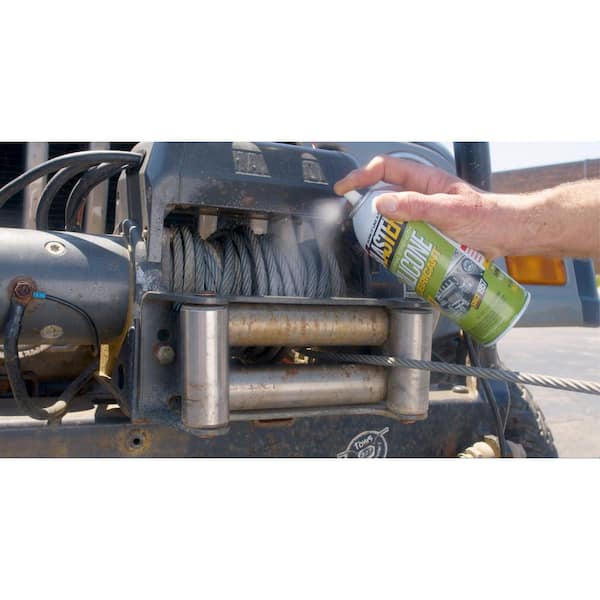This image features the hand of a white male, characterized by a broad wrist and less manicured appearance, spraying a canister of silicone lubricant onto a coiled metal wire rope attached to a winch. The machine, likely a winch, shows signs of age with a gray body and rust patches, including a significant rust spot at the bottom. The rope appears to be thick and may have rust build-up due to its reddish color, suggesting it might be stuck. The canister being used is white with a green label, and the top of the can displays the brand name "Blaster" in bold white and yellow letters on a black background, followed by "Silicone Lubricant" in white and yellow respectively. The image is framed with white bars about two inches thick at the top and bottom, placing the main focus on the central action of lubricating the wire rope.